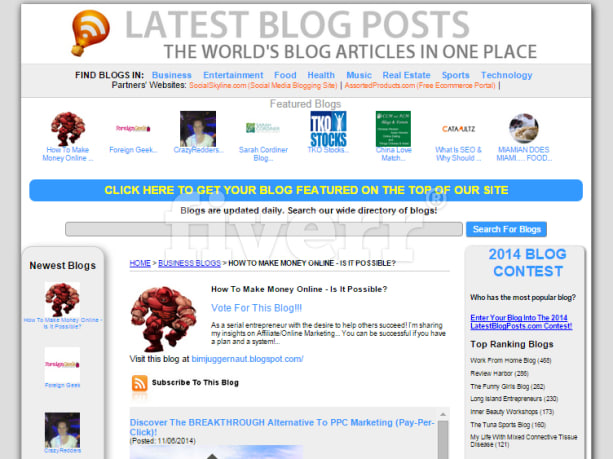The screenshot features a somewhat cluttered website. At the top, large gray text reads "Latest Blog Posts." To the left of this heading is a prominent orange hot air balloon icon adorned with a white Wi-Fi signal. The website's background is predominantly white. Below the title, another heading, "The World's Blog," is displayed, followed by the subtext, "The world's blog articles in one place." 

Underneath this heading is a gray bar extending across the width of the page with the prompt "Find blogs in" followed by blue hyperlinks labeled: Business, Entertainment, Food, Health, Music, Real Estate, Sports, and Technology. 

Further down, the section labeled "Partner Websites" appears in red text. Beneath this section, there is a "Featured Blogs" area showcasing eight thumbnails, each accompanied by blue text names. At the bottom of this section, a blue button with yellow text invites users to "click here to get your blog featured on the top of our site."